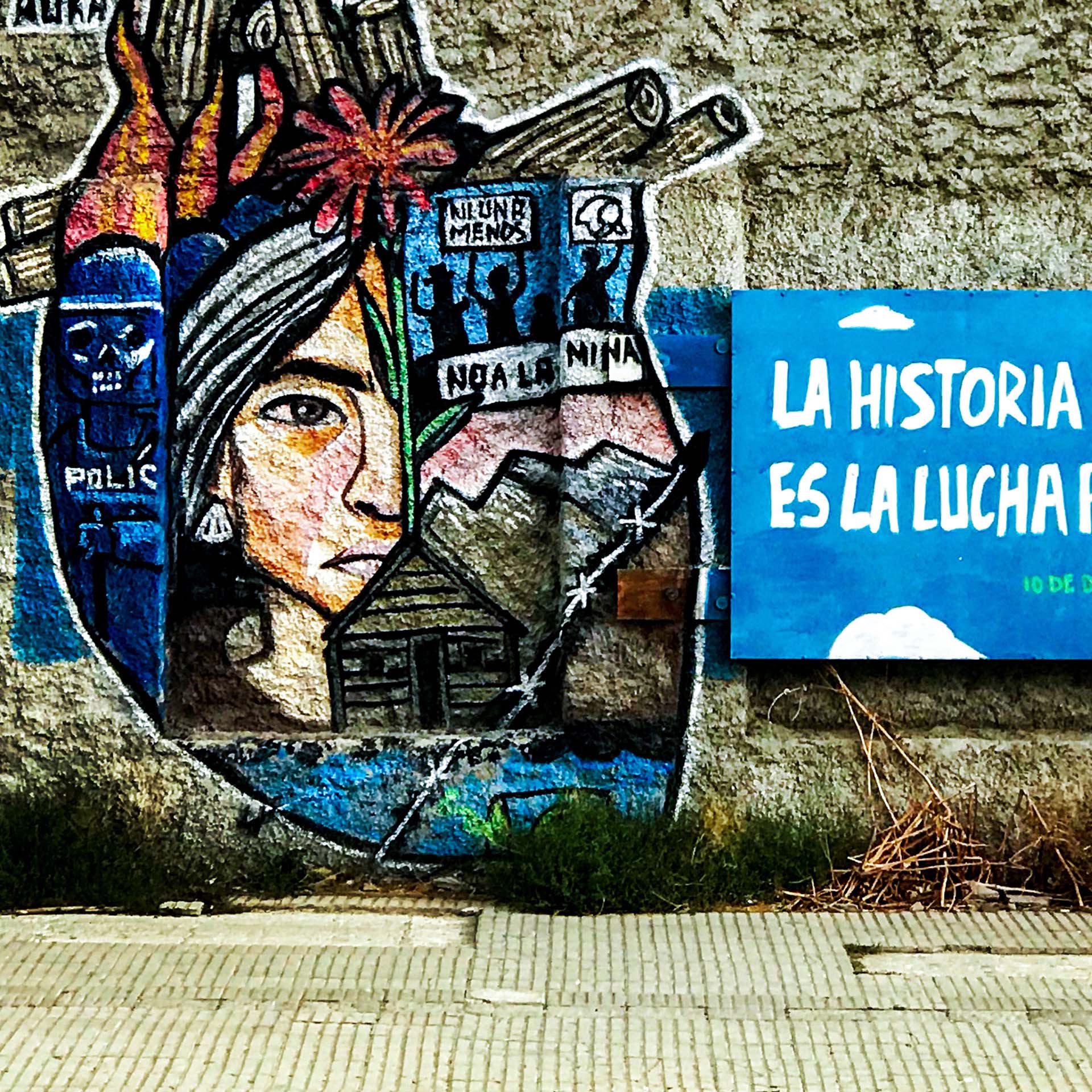The full-color outdoor photograph, taken in natural daytime light, depicts a textured stone wall adorned with intricate graffiti and social art, common in Argentina and reflecting themes of human rights and protest. The lower edge of the square image reveals a cracked and uneven pavement, bordered by a mix of dead and green weeds. A notable blue sign with white text prominently displays the phrase "La Historia Es La Lucha" on the right side. Central and left of the wall features vibrant graffiti, focusing on the shape of a heart filled with compelling imagery: the haunting profile of a native woman's face, a skeletal visage under a helmet bearing the partially spelled word "POLICE," mountains, a small house, symbolic barbed wire, and people engaged in a protest. The mural powerfully intertwines elements of activism and resistance, layered with intricate details that evoke the struggle and resilience of the community.